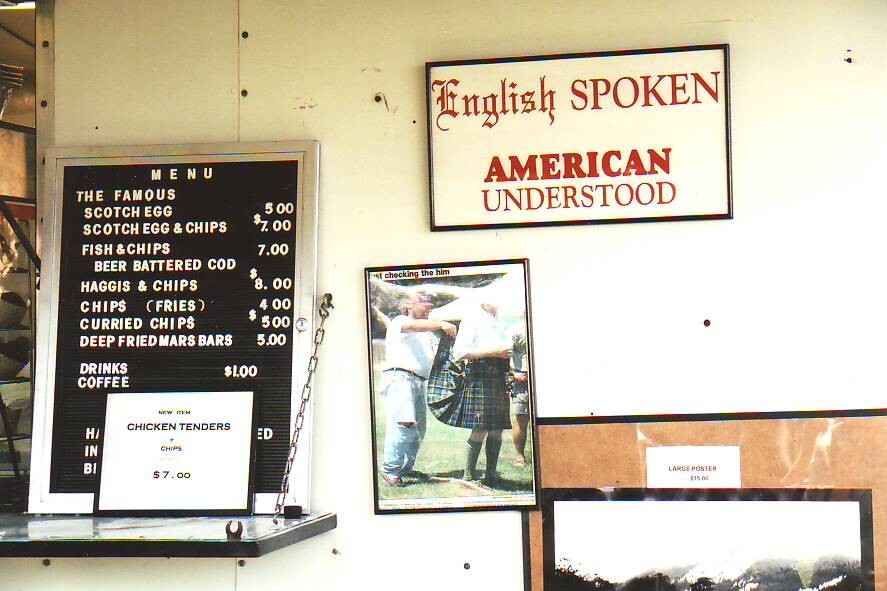This outdoor food service area is captured in a grainy photograph, likely taken with an older camera. The image prominently features a framed sign that declares, "English Spoken, American Understood." Next to it hangs a humorous photo titled "Just Checking the Hymn," depicting a person in a field lifting up the skirt of another individual whose gender is ambiguous. In the bottom right corner, there is another framed item labeled "Large Poster," but any additional details or pricing information are too blurry to discern.

On the left side of the image, a menu showcases an array of offerings, including notable items like the famous scotch egg, scotch egg and chips, fish and chips, beer-battered cod, haggis and chips, chips (fries), curry chips, and deep-fried Mars bars. Additionally, they serve various beverages, with a sign highlighting a new item: chicken tenders plus chips for seven dollars.